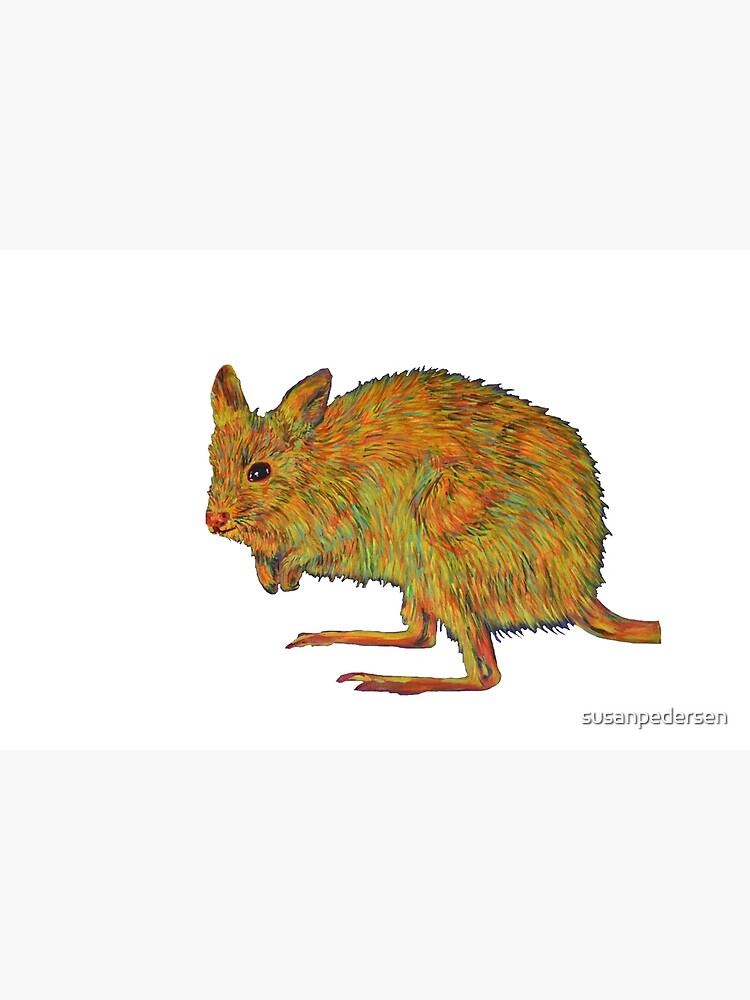This is a detailed color illustration of a small, kangaroo-like creature with characteristics of a mouse and hamster. The animal is depicted in profile facing left, standing on its two long, L-shaped hind legs, with its feet firmly planted on an implied ground against a white background. Its fur is a mix of vibrant red, green, yellow, orange, and turquoise, and appears wiry and spiky. The creature has large, black eyes, an orange-ish to pink nose, and small, pointy ears with orange and black hues. Its face is completely furred, and it has two short arms positioned near its head. A narrow, hairless tail is seen protruding from its back but is cut off by the right edge of the image.